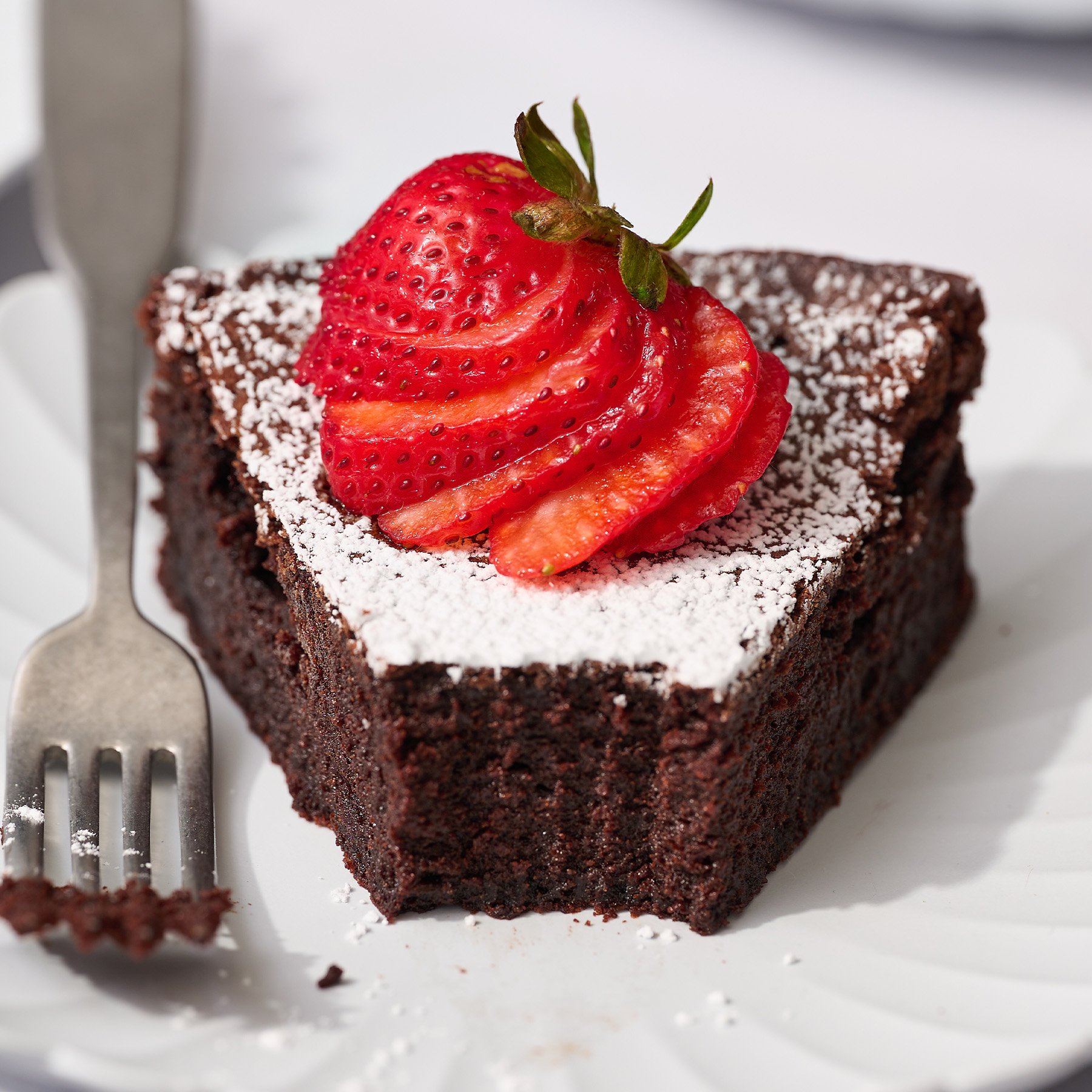The image is a close-up photograph of a triangular slice of dark brown, flourless chocolate cake, elegantly presented on a ridged, white fine china plate. The very tip of the cake has been taken out with the silver fork that rests to the left of the slice. The fork, still covered in remnants of the rich chocolate cake and a dusting of confectioner's sugar, points towards us with its four prongs. The slice of cake is adorned with a sprinkle of white confectioner's sugar on top, creating a delicate contrast. Centered atop the cake is a whole strawberry, finely sliced but still perfectly stacked together, complete with its green stem. The scene is set on a flat, white table, emphasizing the detailed and indulgent presentation of the dessert.